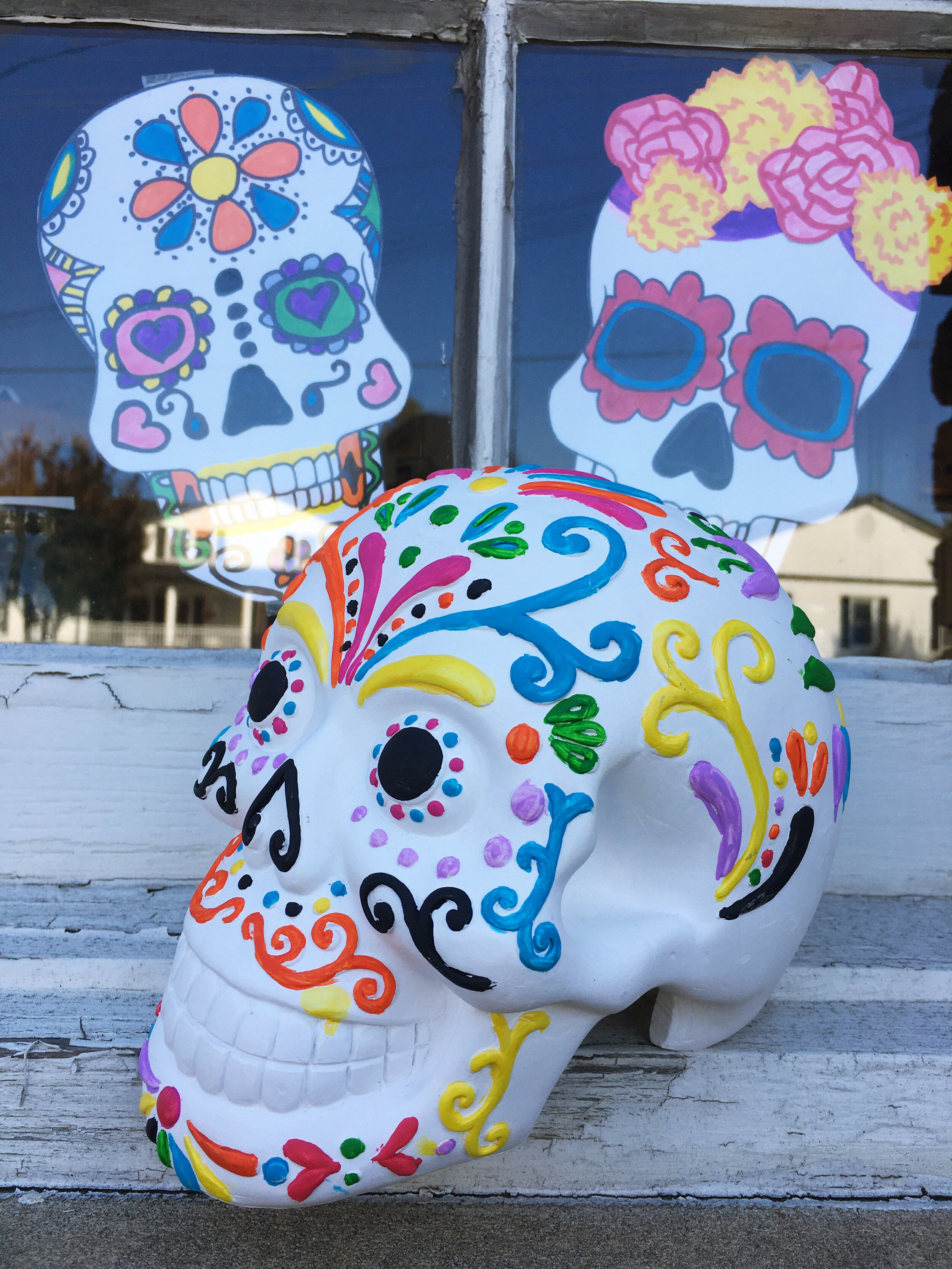The image depicts a richly detailed Day of the Dead scene featuring three sugar skulls. At the forefront, there's a hand-painted ceramic skull resting on a weathered, old barn-style window ledge. This skull is adorned with intricate, swooping designs in vibrant colors including yellow, blue, and pink, highlighted further by black-painted details. The eyes are round and surrounded by pink and blue dots, and yellow ribbons are draped behind the ears. The nose is accentuated by a black pyramid, and an orange curlicue mustache decorates the area above the tightly closed teeth, which are themselves richly painted.

In the background, within the window's panes that are secured with cracked glue and multiple layers of paint, two printed sugar skull images are taped. One represents a female skull adorned with a flower on its head, while the other, presumably male, features various colorful facial designs. The setting suggests a home or a storefront honoring the Day of the Dead, a celebrated Spanish tradition. The combination of hand-painted ceramic and printed skull images, both male and female, creates a harmonious and vividly colored tribute to this festive occasion.